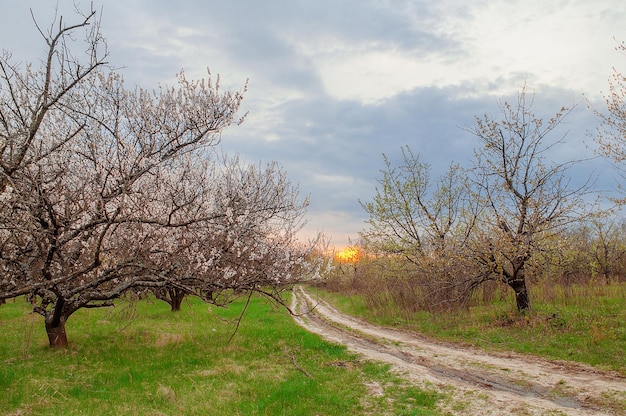The image depicts a serene, rural landscape featuring a dirt trail that appears to have been shaped by vehicle tracks running through the countryside. The trail is flanked by patches of grass, some of which are low-cut while others rise as tall reeds. Trees line both sides of the road, with varying species distinguished by their different shades of leaves. On the left side, there is a notably short tree with wide branches adorned with white-petaled flowers, indicating it might be early spring. The sun is low on the horizon, casting a warm yellow glow and suggesting it is either sunrise or sunset. The sky above transitions from the bright hues of the sun to a lighter, almost blue expanse, partly covered by scattered clouds. The trees on either side of the path appear somewhat barren or just beginning to bloom, which, along with the presence of dry leaves, hints at the chill of early spring or late winter. The overall scene exudes a sense of quiet and timeless beauty, capturing the tranquil essence of the countryside.